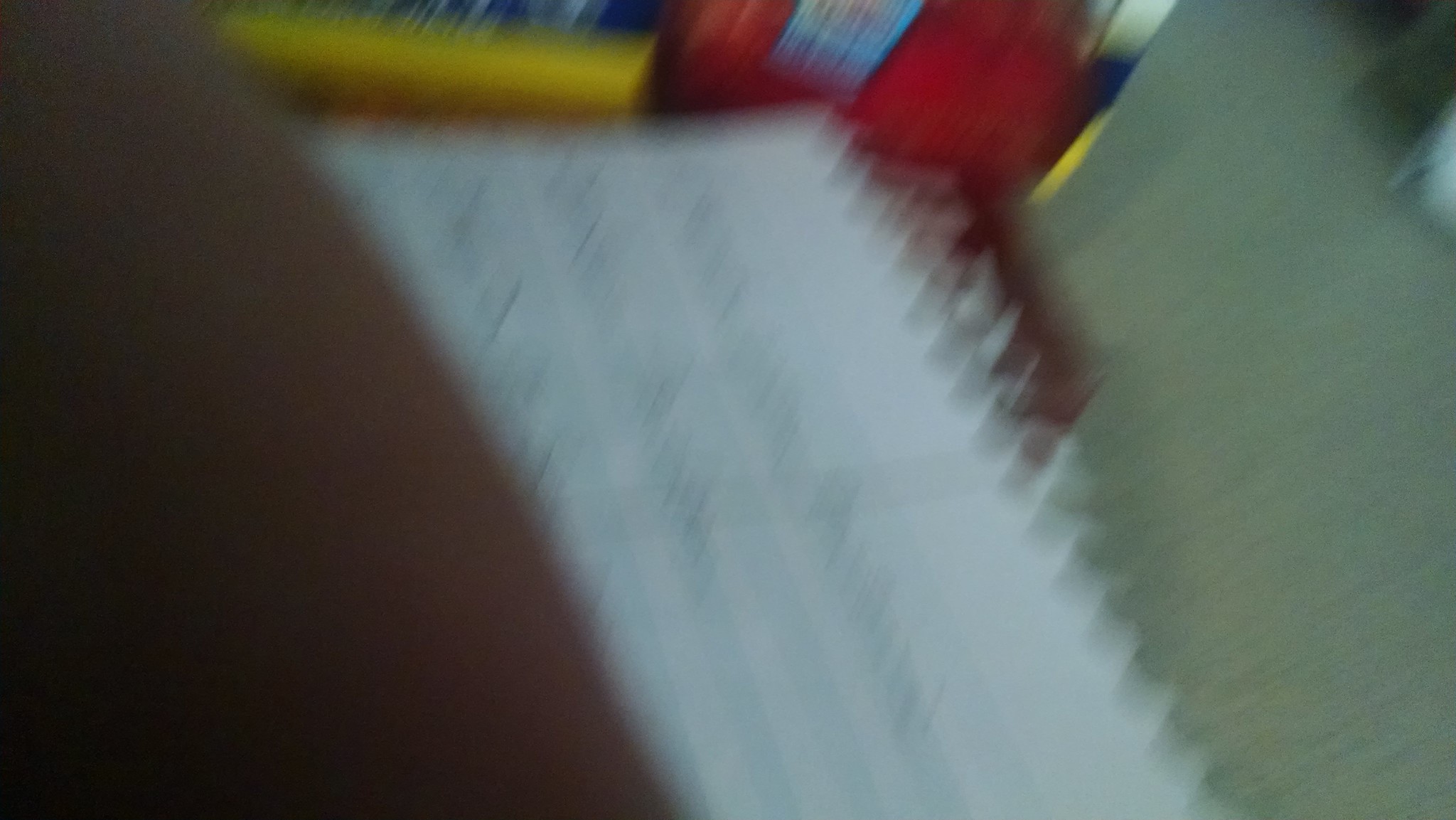This image, captured in a landscape aspect ratio, is characterized by significant motion blur, obscuring the details of its subjects. On the left side, there is a smudge with a light skin tone color that is difficult to distinguish. Central to the image is a white rectangle with illegible scribbling on it, and its ragged edges suggest it is a piece of notebook or binder paper that has been torn out. The right side of the frame features a grayish-green area, likely a carpet, adding to the indistinct nature of the photo. Near the top, a red shape is visible alongside a box with a touch of yellow, contributing to the overall confusion and lack of clarity in the image.